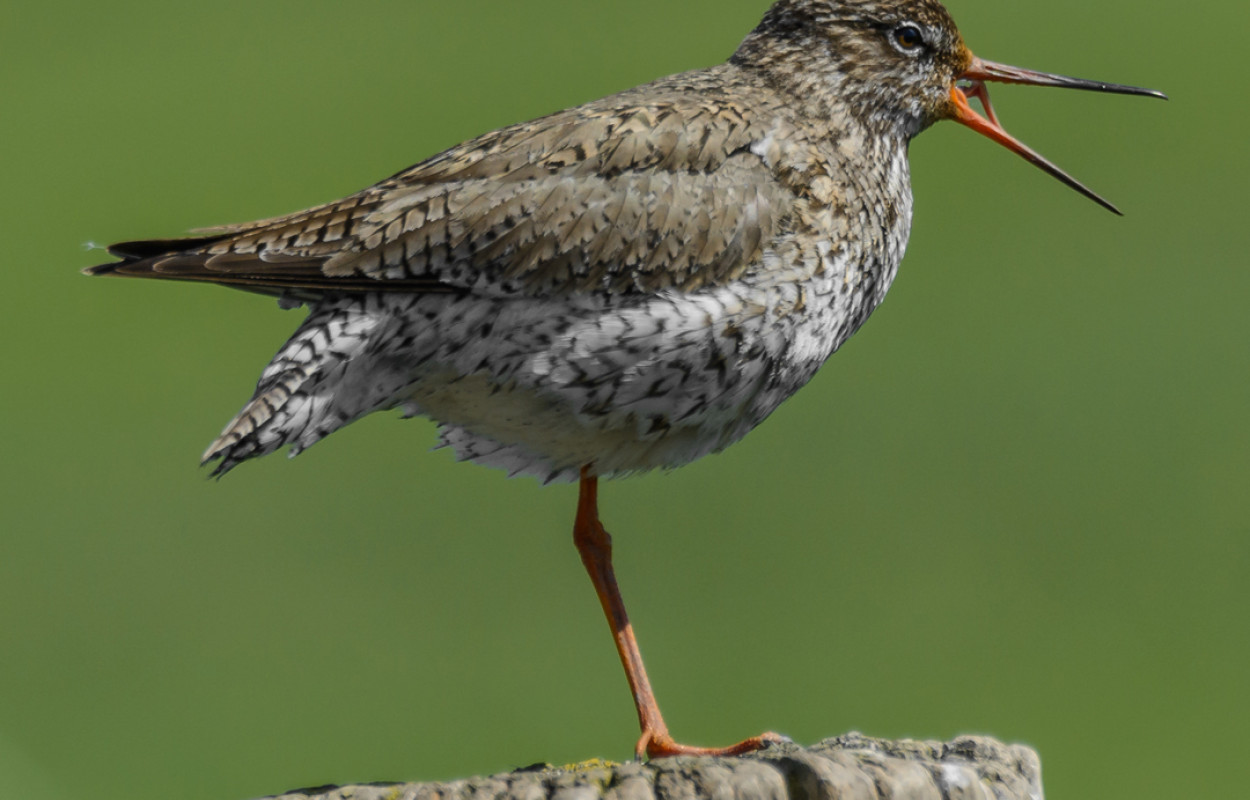The photograph captures a small bird in a side profile view, standing on one leg atop a piece of wood or rock against an olive green background. The bird's beak is open, displaying its tongue – an unusual sight. The beak is long and multicolored, transitioning from black at the tip, to dark orange, and finally to yellow closest to the body. The bird’s plumage is predominantly pale gray with darker brownish-gray patterns on its wings, and it has a white underside with some black streaks. It has beady brown eyes and short tail feathers that match the color of its body. The bird's other leg is either tucked up within its feathers or missing. The scene is reminiscent of a beach-dwelling bird known as a snowbird, although it also bears resemblances to species such as a blue jay or small cardinal.